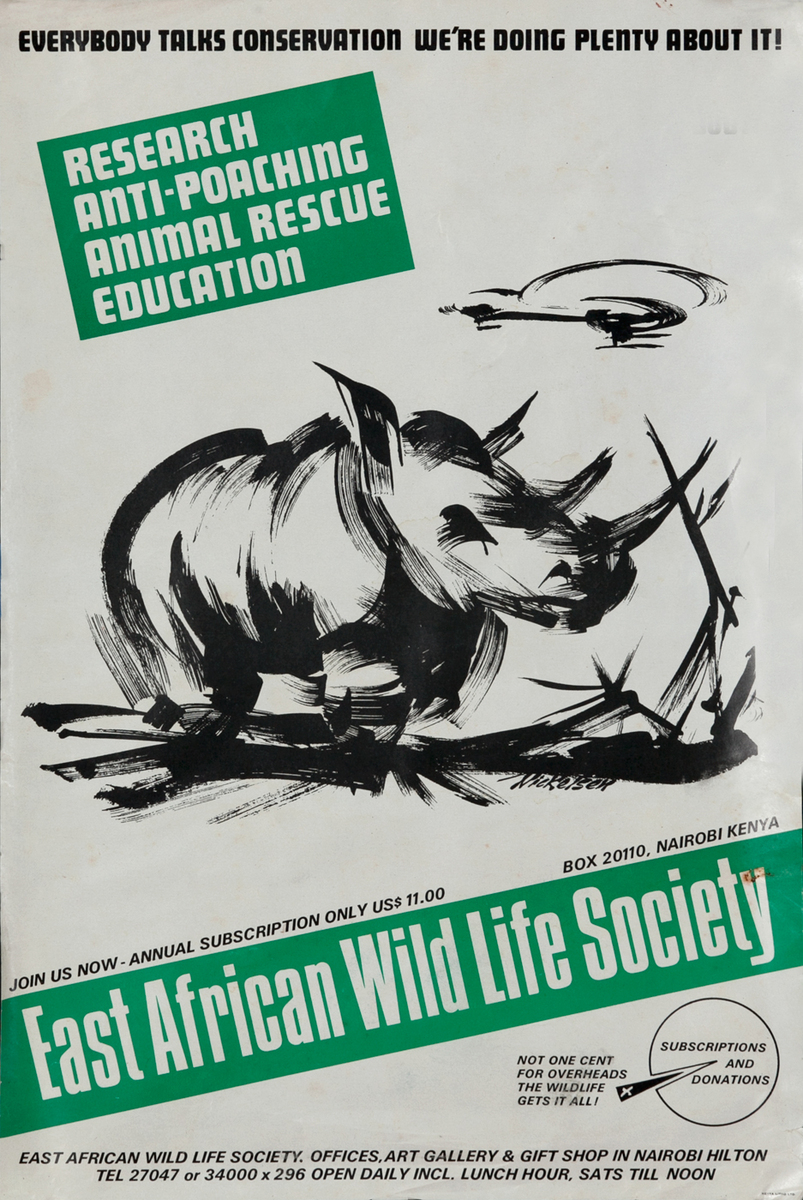The front cover of the flyer for the East African Wildlife Society features a prominent, sketch-like drawing of a two-horned rhinoceros with a helicopter flying above it. The header at the top of the flyer reads, "Everyone talks conservation—we're doing plenty about it!" in black text. Below this, a green box with white text lists the Society's key initiatives: "research, anti-poaching, animal rescue, education." Underneath the green box is the rhino illustration, which includes detailed features like long ears and hair on its forehead, with the artist's name in black cursive next to it. Further down, the flyer invites readers to "join us now," advertising an annual subscription for only $11 USD, directed to a P.O. Box in Nairobi, Kenya. Another green box, spanning the width of the cover, states, "East African Wildlife Society—not one cent for overheads, the wildlife gets it all." Additional details include subscription and donation information, and contact details for the Society's offices, art gallery, and gift shop located in the Nairobi Hilton. The flyer emphasizes that all contributions go directly to wildlife conservation efforts.